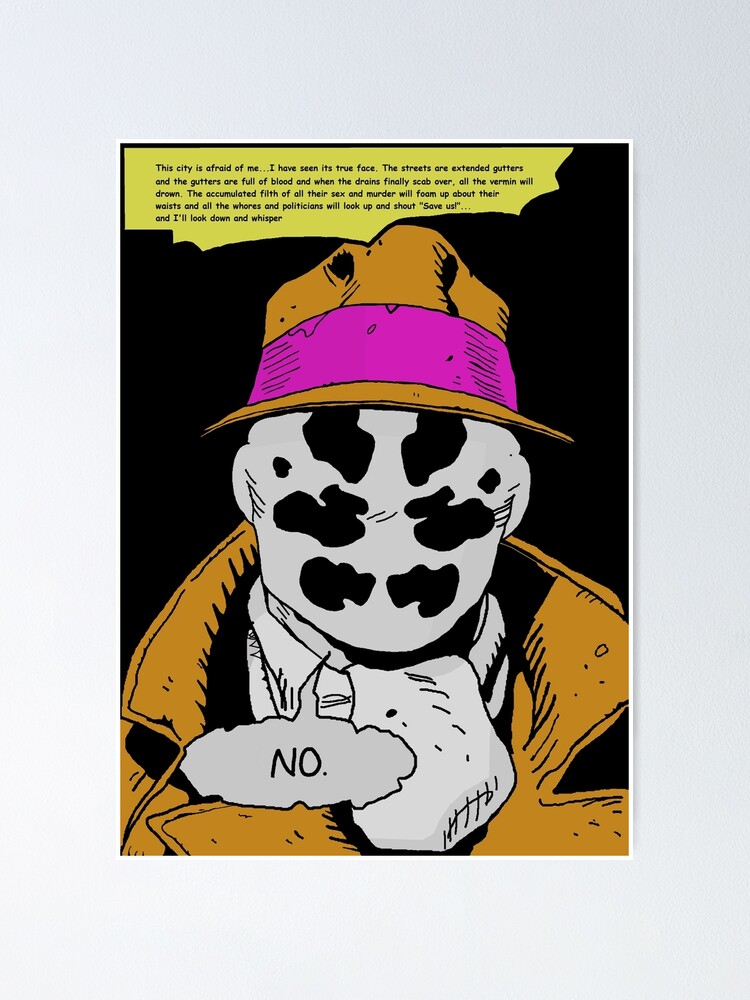The image is a comic-style depiction of a faceless man viewed from the chest up. He's adorned in an orange trench coat and an orange bucket hat with a fuchsia stripe around its middle. His skeletal face is white with black shadowing for eyes and mouth, marked by six different-shaped holes. The background is black, and a speech bubble near his mouth contains the word "No." Above him, in a yellow section with black text, reads a monologue: "This city is afraid of me. I have seen its true face. The streets are extended gutters, and the gutters are full of blood. And when the drains finally scab over, all the vermin will drown. The accumulated filth of all their sex and murder will foam up about their waist, and all the whores and politicians will look up and shout, 'Save us.' And I will look down and whisper, 'No.'" The scene suggests a dark, adult-themed comic book setting.